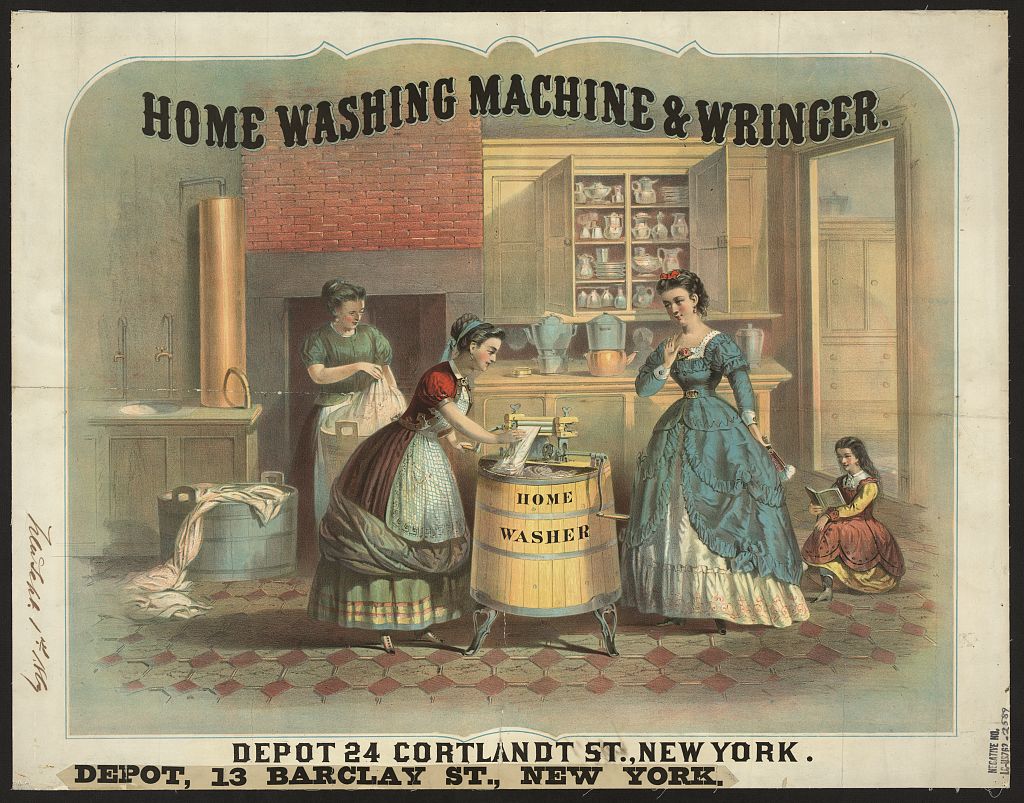This detailed image showcases a vintage advertisement for a home washing machine and ringer. The ad, depicted through a drawing or painting, is framed with a black border and a cream-colored matte border. Central to the image is an early manual washing machine resembling a barrel, equipped with a hand-cranked ringer on top. 

In the scene, multiple women are engaged in laundry tasks. On the left, a middle-aged woman dressed in a red dress with a green skirt underneath and a white apron is actively washing white clothes. To the right, another woman, adorned in an elegant blue ball gown with a white skirt underneath, observes the washing process. Further right, a young girl in a brown-red dress sits on the floor, engrossed in reading a book. In the background, perhaps reflecting a more affluent household setting with visible cabinets and fine china, a woman in a green shirt is either folding or bagging up laundry. 

Prominent black font at the top of the image reads, "Home Washing Machine and Ringer," while the bottom provides an address: "DePaul 24, Courtland Street, New York, Depot, 13 Barclay Street, New York."